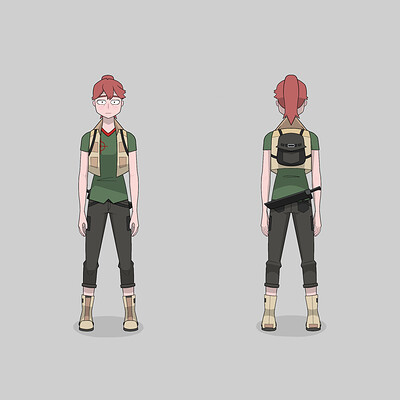In this cartoon-style illustration, the character is shown from both the front and back perspectives side-by-side. The figure has distinctive red cartoon hair that flows over her face but doesn’t cover her wide eyes, which have dots for pupils, and her pale white skin. Her facial expression suggests a vacant or blank stare. She is dressed in a green t-shirt with red trim around the neck, and over it, she wears a short khaki-colored vest with pockets on either side. Her outfit includes black cargo-style pants with pockets on the sides and back, and tan combat boots with yellow stitching and laces up the front.

From the back view, her red hair is tied up in a ponytail. She carries a small black backpack and a sheathed combat knife clipped onto the back of her pants. The background of the image is a flat light gray color, adding to the focus on the character's detailed attire and features.